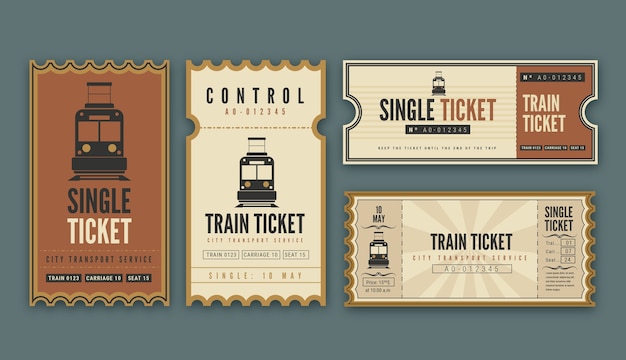This is an advertisement mock-up showcasing various types of train tickets in a visually striking graphic arts design. The composition features four distinct tickets arranged against a gray background, with a color palette of brown, beige, and olive. The tickets vary in orientation: the two on the left are vertical, while the two on the right are horizontal.

The first vertical ticket on the left is dark red rust-colored with a unique punched-notch design for easy tearing. It bears the label "Single Ticket" and includes an image of a train, along with partial details like "City Transport Service," "Train Number," "Carriage Number," and "Seat 15." 

Next to it is another vertical ticket labeled "Control AD," mentioning the "10th of May," and sporting similar train and seating information. 

To the right, the horizontal tickets mirror the vertical ones in design and information, but differ in orientation. The combination of black, brown, and beige lettering enhances readability and aesthetic appeal.

This well-constructed advertisement represents different types of train tickets, combining detailed visuals and textual elements to create a comprehensive promotional graphic.